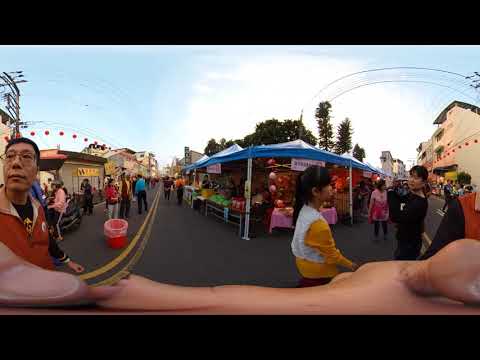This image captures a lively outdoor street market, likely in China or Japan, set in a bustling downtown area. The market spans an asphalt road, distinguished by a double yellow line down the center. Blue tents line both sides of the street, hosting an array of stalls selling souvenirs, food, fruits, and produce like red and green items. Decorative red, balloon-like lights dangle overhead, adding a festive touch. White and yellow signs with unreadable text adorn some stalls, while strings of lights crisscross the street, illuminating the scene against a partly cloudy sky.

In the foreground, a stall on the right side of the street displays produce and possibly balloons. Adjacent to it, a card table with a pink tablecloth adds to the eclectic mix. Prominently in view is a woman in a yellow sweater with a white vest, standing near a man in a red jacket and glasses. The street, busy with people in colorful attire—black, red, yellow—is alive with activity. Some individuals are seated, engaged in conversation, while others wander leisurely amid the market stalls. Overhead, telephone lines stretch across the scene, encapsulating a typical, vibrant summer evening at an Asian street fair.